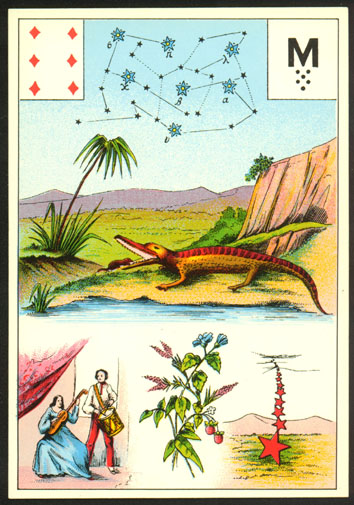This image resembles an intricately designed vintage card poster, potentially of native Mexican origin. It features a sophisticated border composed of a thick black frame, followed by a white frame, and finishing with a thin black line.

In the upper left-hand corner sits an arrangement of six red diamonds, akin to those on a playing card, with three diamonds aligned in a row next to each other. On the right-hand side of the poster, there is a bold black letter "M," positioned above a formation of six dots: five dots arranged like the number five on a dice, with an additional dot centered below them.

The poster showcases a constellation, adorned with blue flowers interspersed among the stars and connected with thin lines. Below the constellation, mountains, cliffs, and a body of water—either an ocean or river—provide a natural backdrop. A dinosaur or lizard and a solitary palm tree enhance the scenic detail.

In the lower section, a scene captures a woman playing a guitar and a man playing a drum, framed by a vivid red curtain to the side. Nearby, a distinctive flower with blue petals and red berries adds a touch of color. The image further features a photograph of stars depicted as falling from the sky, rendered in striking red hues as they descend towards the earth.